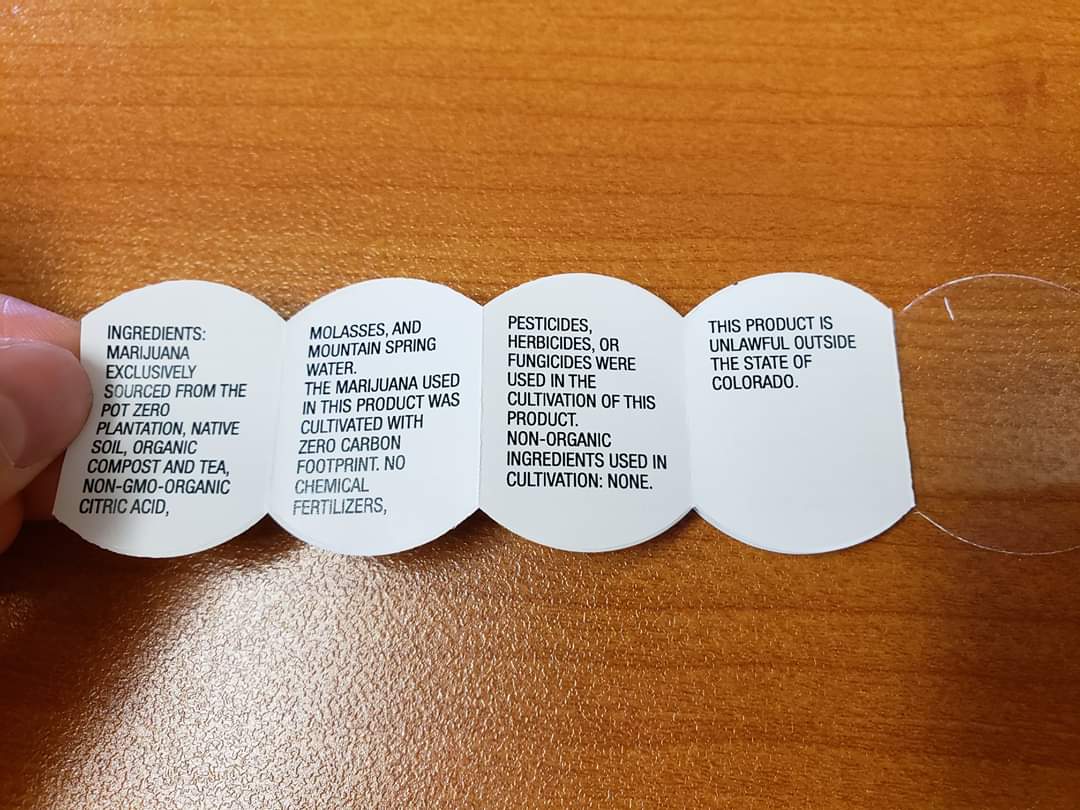The image is a rectangular photograph featuring a hand holding a small, folded, white pamphlet with black text. The pamphlet appears to be a product label for legal marijuana, sourced exclusively from the Pot Zero Plantation in Colorado. It unfolds into four vertical, dog tag-shaped panels, which are spread out and display a detailed description of the product's cultivation and ingredients. The person holding the pamphlet is visible on the far left side of the image, with their thumb and the top part of their index finger ensuring the label stays open. The text on the pamphlet highlights that the marijuana was grown with zero carbon footprint and without the use of chemical fertilizers, pesticides, herbicides, or fungicides. It lists ingredients including native soil, organic compost, tea, non-GMO organic citric acid, molasses, and mountain spring water, all ensuring the product's purity and organic quality. Additionally, it notes that the product is unlawful outside the state of Colorado. The scene is set against a light brown, walnut-stained wooden tabletop, emphasizing the natural theme of the product.